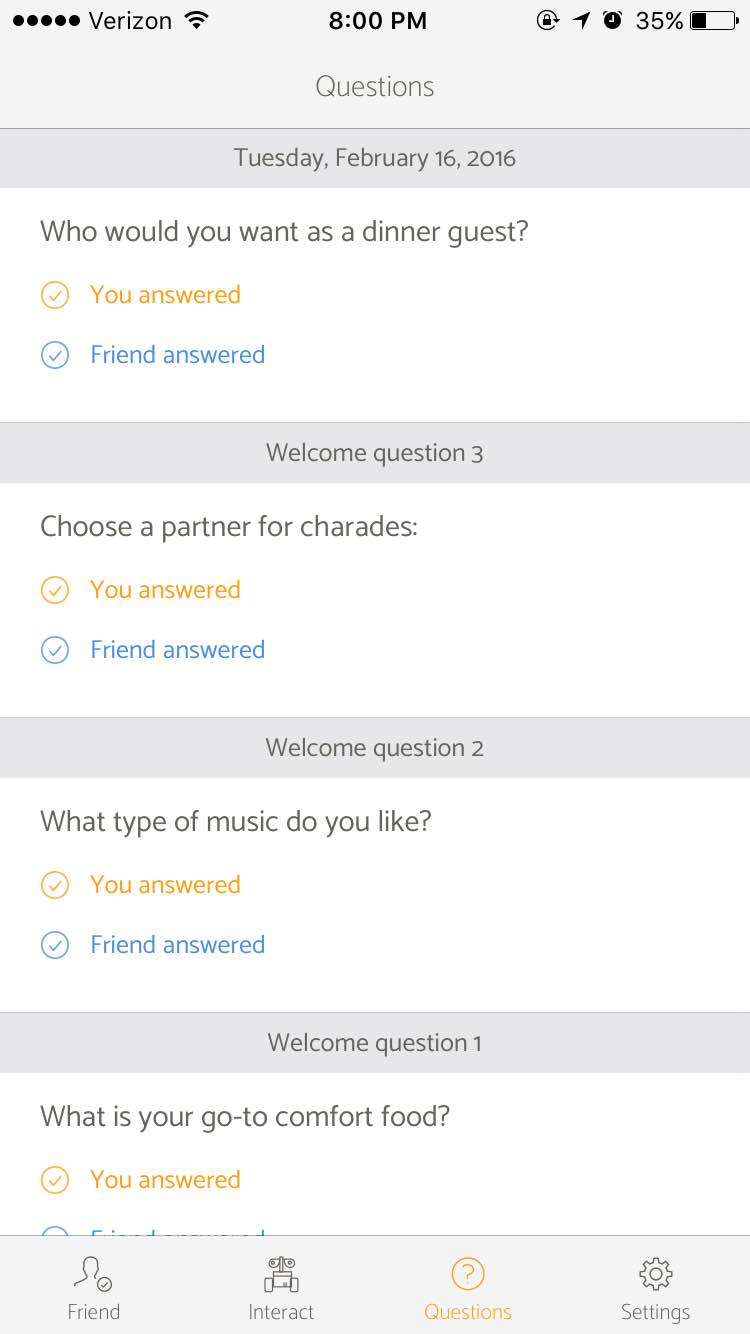A smartphone screen displays a conversation between two friends on a questionnaire app at 8:00 PM. The phone has a Verizon signal with full bars but only 35% battery life remaining. In the light grey box at the top, it indicates "Questions Tuesday February 16th." Below this, in a darker grey box, a series of questions and answers is shown:

1. "Who would you want as a dinner guest?" with answers from both users.
2. "Choose a partner for charades," also showing responses from both.
3. "What type of music do you like?" with the users' preferences noted.
4. "What is your go-to comfort food?" includes both users' comfort food choices.

At the bottom of the screen, there are options available: "Friend," "Interact," "Questions," and "Settings." The app interface effectively captures their interaction across multiple queries.